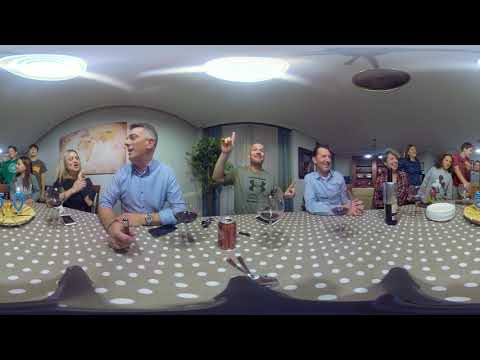In this low-resolution, slightly warped 360-degree photograph, we see a lively family gathering taking place in a cozy, bright room with white walls and pot lights in the ceiling. The room is decorated with blue and white curtains and a few pictures on the walls, including a map painting. A large table, covered with a brown tablecloth adorned with white polka dots, is the focal point, strewn with various items such as mobile phones, cans of pop, empty wine glasses, and paper plates.

Starting from the left side of the table, three people are visible in the background. Of these, two individuals with short hair—one in a green shirt and the other in a brown shirt—are standing. Sitting at the table in front of them is a girl with long brown hair, wearing a gray shirt. Beside her, a blonde woman in a dark blue shirt turns her attention to a man in a light blue collared shirt, who sits slightly off-center to the right. This man, with gray hair, is holding something in his hand.

To the right of this man, another man in a gray Under Armour shirt raises his right hand with one finger extended. Further to the right is a dark-haired man sitting at the table, dressed in another blue collared shirt. Next to him sits a woman with dark brown hair in a red patterned shirt.

Continuing to the right, another woman with long dark brown hair, wearing a blue shirt, stands, while a girl in a Mickey Mouse patterned gray shirt and a boy in a red shirt complete the group.

Everyone in the picture is engaged, smiling, and interacting, creating a festive and joyful atmosphere reflective of a family get-together or party.